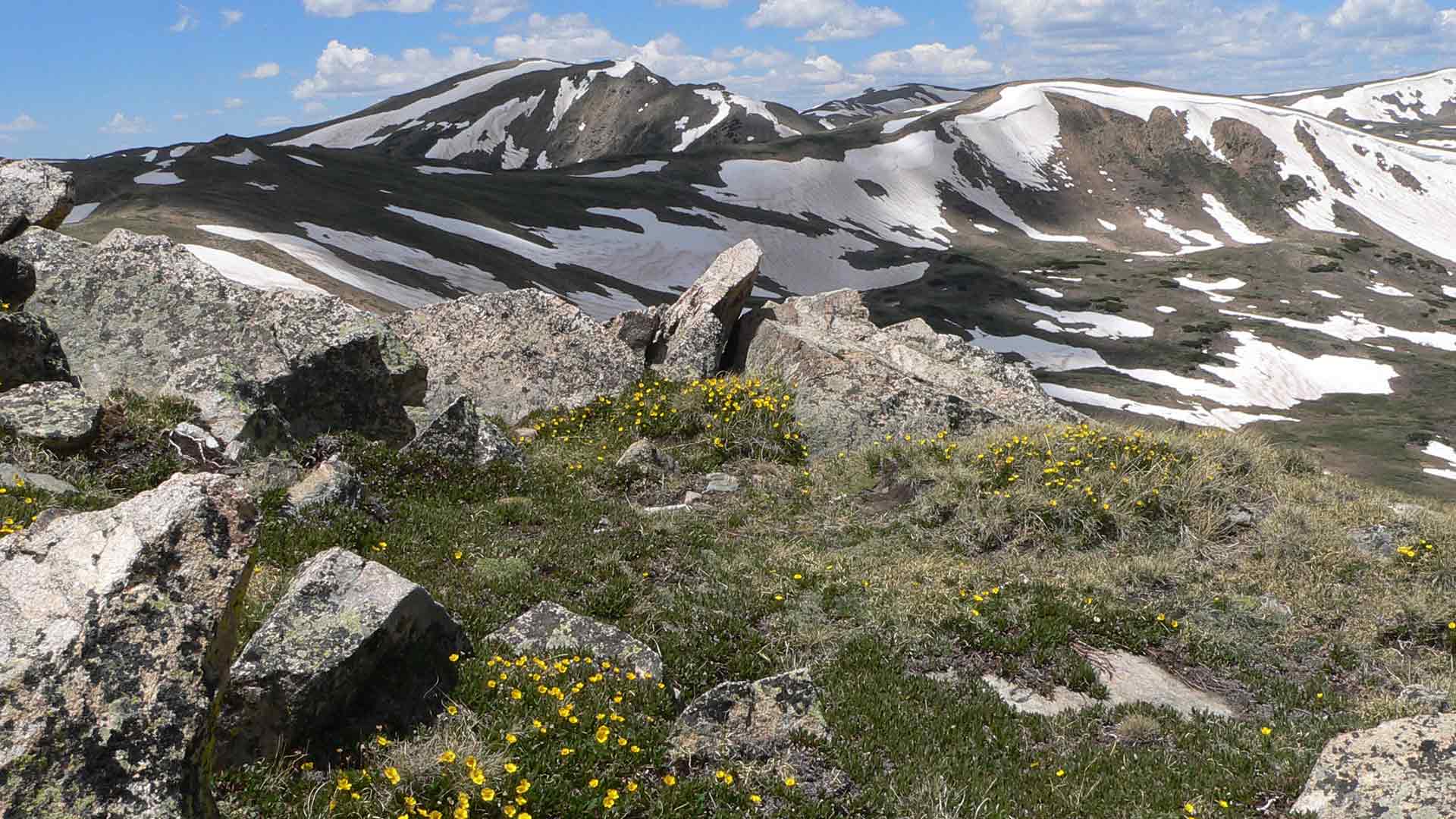This photograph captures a stunning mountain landscape during the daytime, oriented in a landscape format. The scene is dominated by a prominent gray mountain in the background, featuring dark gray and brown slopes with scattered patches of melting snow in its crevices, giving hints of early spring. Above the mountain, the sky is a vibrant blue, adorned with wisps of white clouds. 

In the foreground, large, jagged gray rocks with pink and black hues, possibly granite, are prevalent. These rocks are interspersed with patches of short green grass and clusters of small yellow wildflowers, indicating the warming weather. The bottom half of the image offers a detailed view of these rugged rocks and delicate flora, creating a rich contrast against the imposing mountain in the distance. Together, these elements create a harmonious composition that captures the serene yet dynamic essence of this natural landscape.